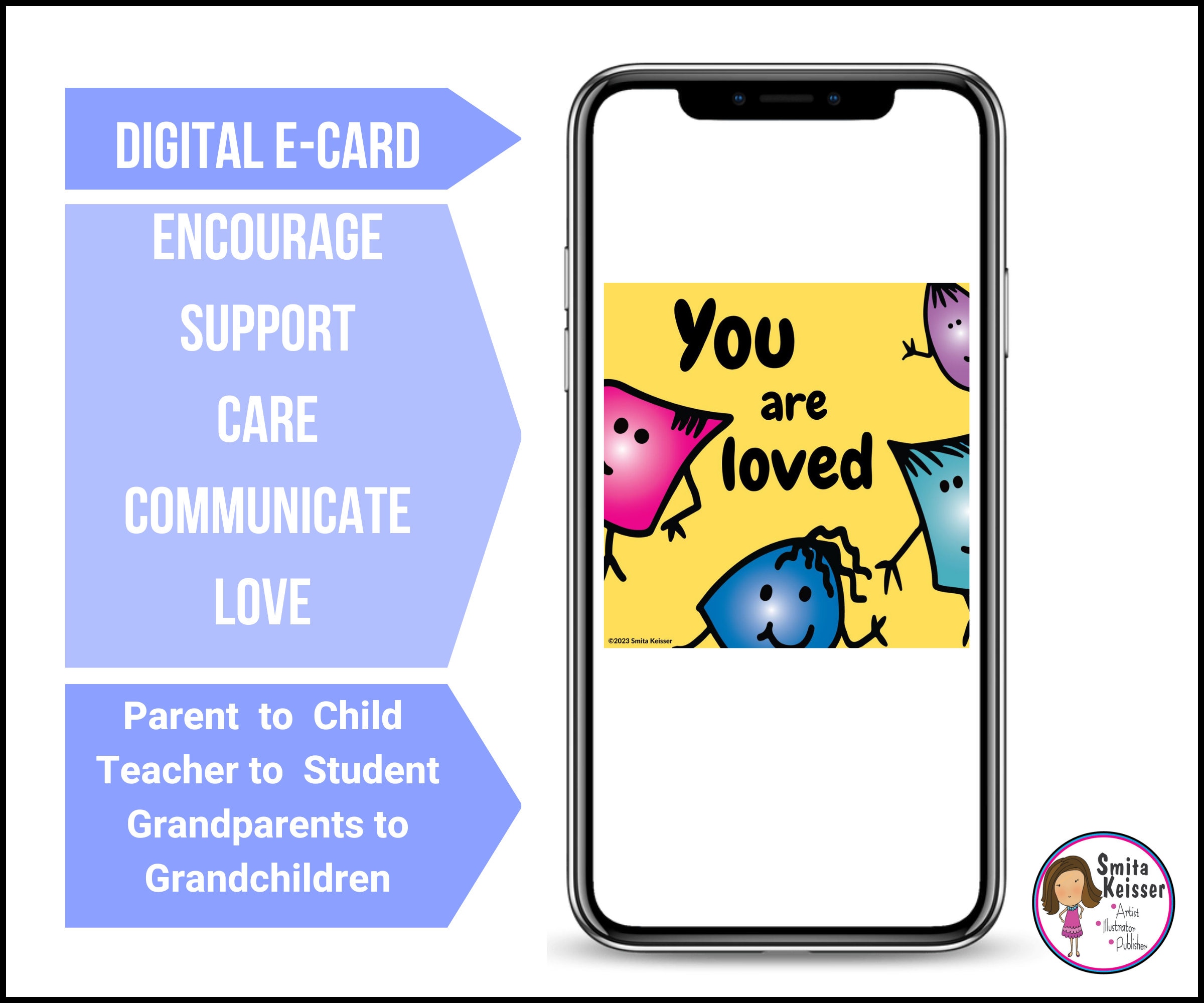The image features a white background with an array of colorful elements on the left side and a drawing of a smartphone on the right. On the left, there are three pentagonal shapes with white text on a purple background, listing the words "digital e-card," "encourage," "support," "care," "communicate," and "love." Below these shapes, it says "parent to child," "teacher to student," and "grandparents to grandchildren." Each phrase points towards a black-edged smartphone on the right. The smartphone has a yellow screen with the message "You are loved" and displays four small, colorful shape characters with smiling faces—a blue face, a pink face, and two purple faces. Surrounding these elements are various smaller shapes in light blue, purple, and pink. In the bottom right corner of the image, there is a small circle featuring a drawing with the name Smita Kaiser, the artist who created the piece.